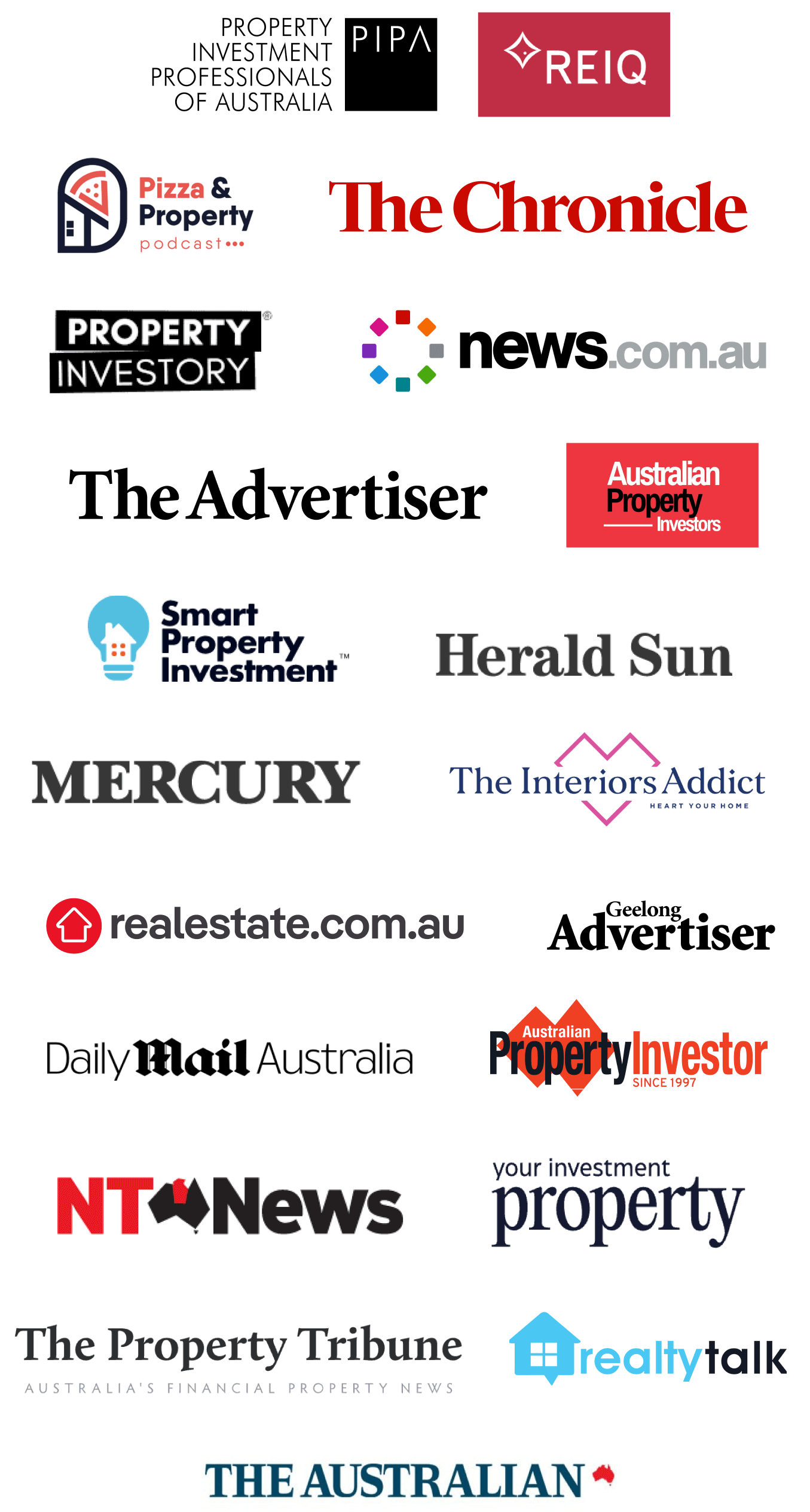The image, set against a pristine white background with no border, displays a vertically arranged list of sponsors for a company, likely affiliated with property investment. At the very top, bold black ink spells out "Property Investment Professionals of Australia," adjacent to which is a black box featuring white letters that read "PIPA" for the Property Investment Professionals Australia.

To the right, within a wine-colored rectangular box, white capital letters spell out "REIQ," complemented by a small white diamond shape. Below, on the left, "Pizza and Property Podcast" is denoted alongside their distinctive black, white, and red logo, featuring a pizza slice.

To the right of this, "The Chronicle" is displayed in red lettering. Below, on the left side, the words "Property" and "Investoree" appear inside two separate black boxes. "Property" is highlighted in bold white letters, while "Investoree" is rendered in thinner white capital letters.

On the right, "news.com.au" is presented, with "news" in bold, black, lowercase letters and ".com.au" in smaller, gray, lowercase letters. Adjacent to the word "news" is a circle composed of tiny, multi-colored squares in shades of red, orange, purple, blue, green, and turquoise.

Below, on the left, "The Advertiser" is written as a single word. To the right, a red box encloses the text "Australian Property Investors," with "Australian" and "Investors" in white text and "Property" in black text. The list continues further down the page with additional sponsors, predominantly consisting of property investment and news sources.